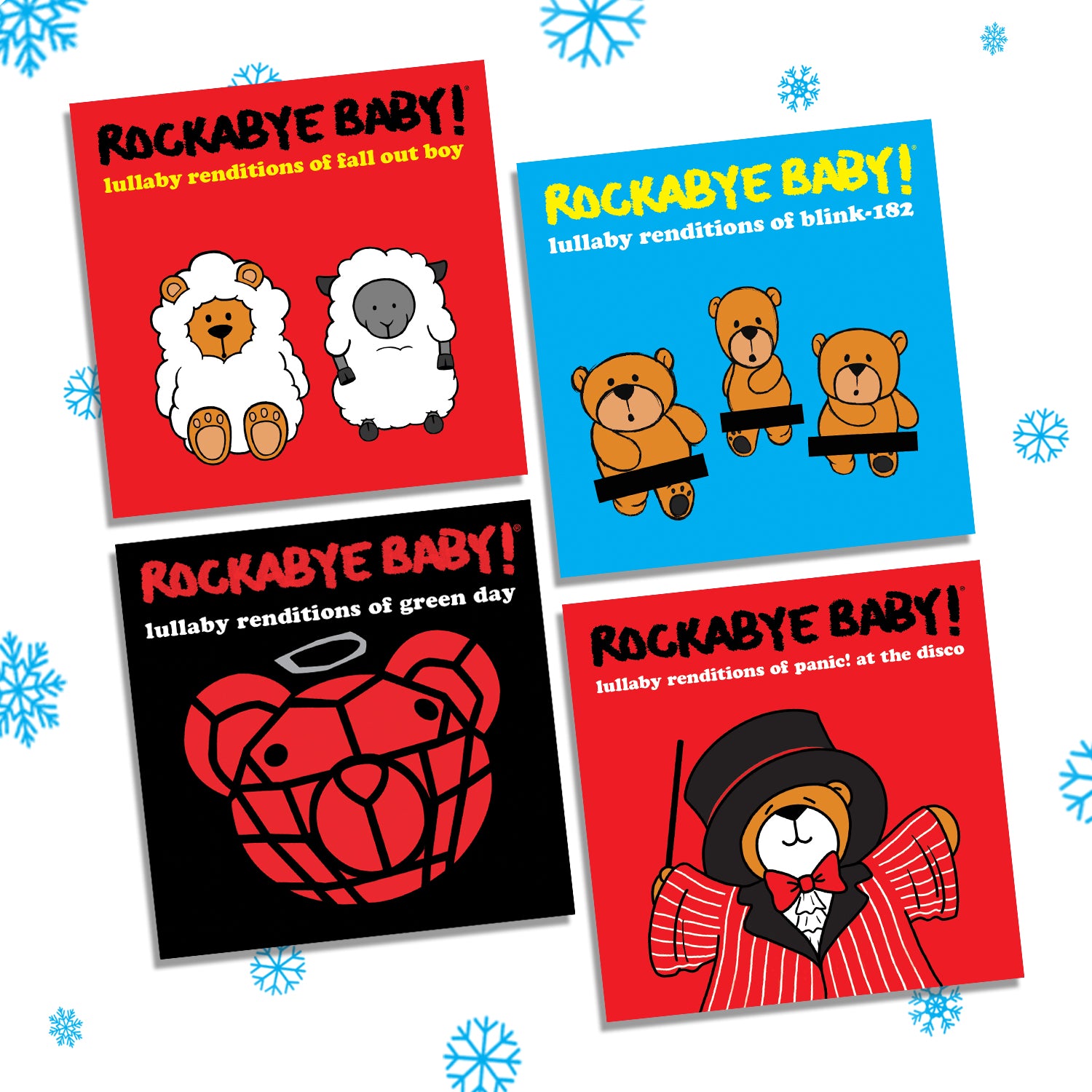The image showcases four square album covers against a white background adorned with small blue snowflakes. The squares are arranged at a slight diagonal angle, with the top right corner elevated. The squares are positioned next to each other and stacked, creating a neat grid pattern. 

- **Upper Left Square (Red Background)**: This cover features a red backdrop with the title *"Rockabye Baby"* written in black at the top. Below that, in yellow, it reads *"Lullaby Renditions of Fall Out Boy."* The illustration depicts two sheep; one appears to be a bear disguised as a sheep, while the other resembles a gray dog in sheep's clothing.

- **Upper Right Square (Blue Background)**: This cover stands out with its blue background. The title *"Rockabye Baby!"* is boldly written in yellow at the top, followed by *"Lullaby Renditions of Blink-182"* in white beneath it. The bottom features three teddy bears, each bearing a small black rectangle on their lower abdomen.

- **Lower Left Square (Black Background)**: Against a black background, the title *"Rockabye Baby!"* is prominently displayed in red at the top. Below, in white, the text reads *"Lullaby Renditions of Green Day."* A large red bear head takes center stage, featuring a gray halo and thick black lines dividing its face into sections.

- **Lower Right Square (Red Background)**: This cover, set against a red backdrop, displays *"Rockabye Baby!"* in black at the top. Below, in white, it states *"Lullaby Renditions of Panic! At The Disco."* An illustration of a bear dressed in a red jacket with white stripes, a red bow tie, and a black hat with a red band around its base, extends its arms out to the sides.

Each album cover is vividly colored and artistically designed to reflect the theme of lullaby renditions of famous rock bands.